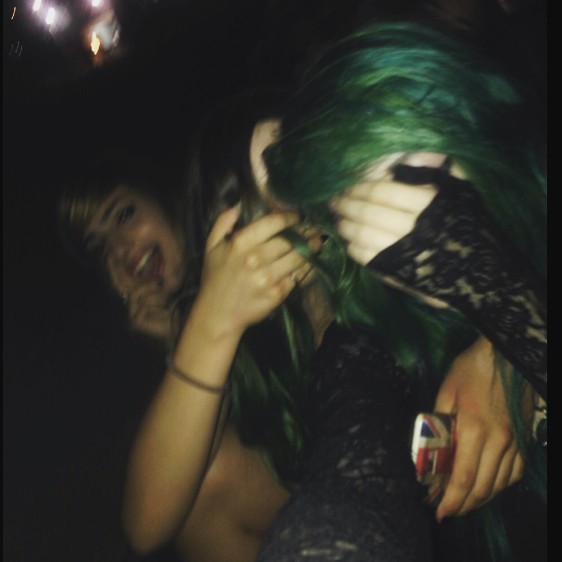This photograph, taken at night and slightly blurry, captures a candid moment featuring three young girls, likely in their teenage years to early twenties. The girl on the far left has dirty blonde hair, is smiling broadly, and appears to be caught in a moment of surprise or delight. She is the only one fully visible. The girl in the middle has dark brown hair and is partially obscured as she covers her face with her hand. The girl on the right, with a mix of light and dark brown hair, is also covering her face with her hands, possibly in laughter. Both the girl in the middle and the girl on the right exhibit playful, shy gestures. The girl on the right is wearing a black shirt with lacy long sleeves. Notably, the middle girl is holding a phone with a British flag design on its back. The photo suggests an outdoor setting, likely illuminated by a flash, rendering the background indistinguishable. The overall ambiance hints at a post-party or celebratory moment among friends.